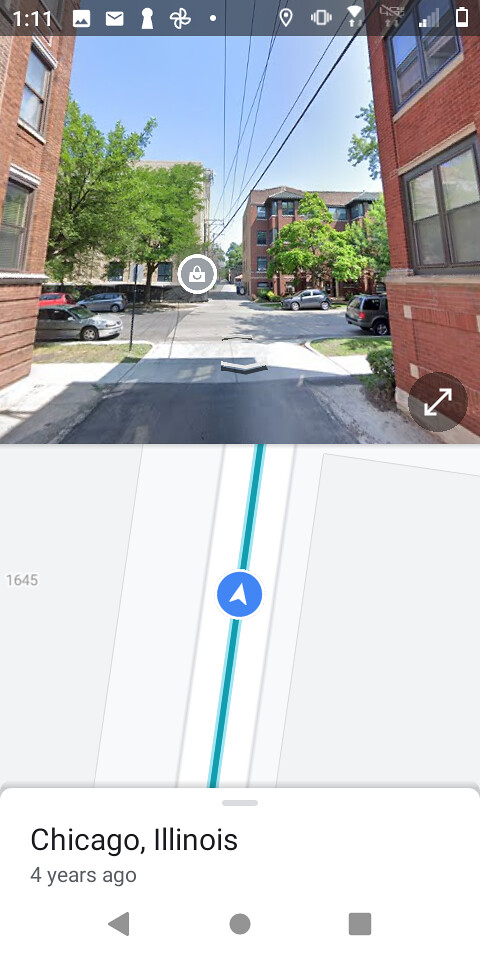The image depicts a once-functional navigation room located in the lower section, specifically indicating "Chicago, Illinois." Four years prior, an airplane departed, leaving behind a complex array of symbols. A prominent gray circle is displayed alongside a large gray square. At the top, the number "1,111" is prominently featured, followed by another square, a mountain symbol, and a letter. The right side reveals a fan shape with a dot and a space in-between, alongside a pin and a vibrating square. Central to the image is a street lined with green-leafed trees, with vehicles parked along the road. The far left side showcases a large building, while the right side of the image is dominated by vibrant red tones.